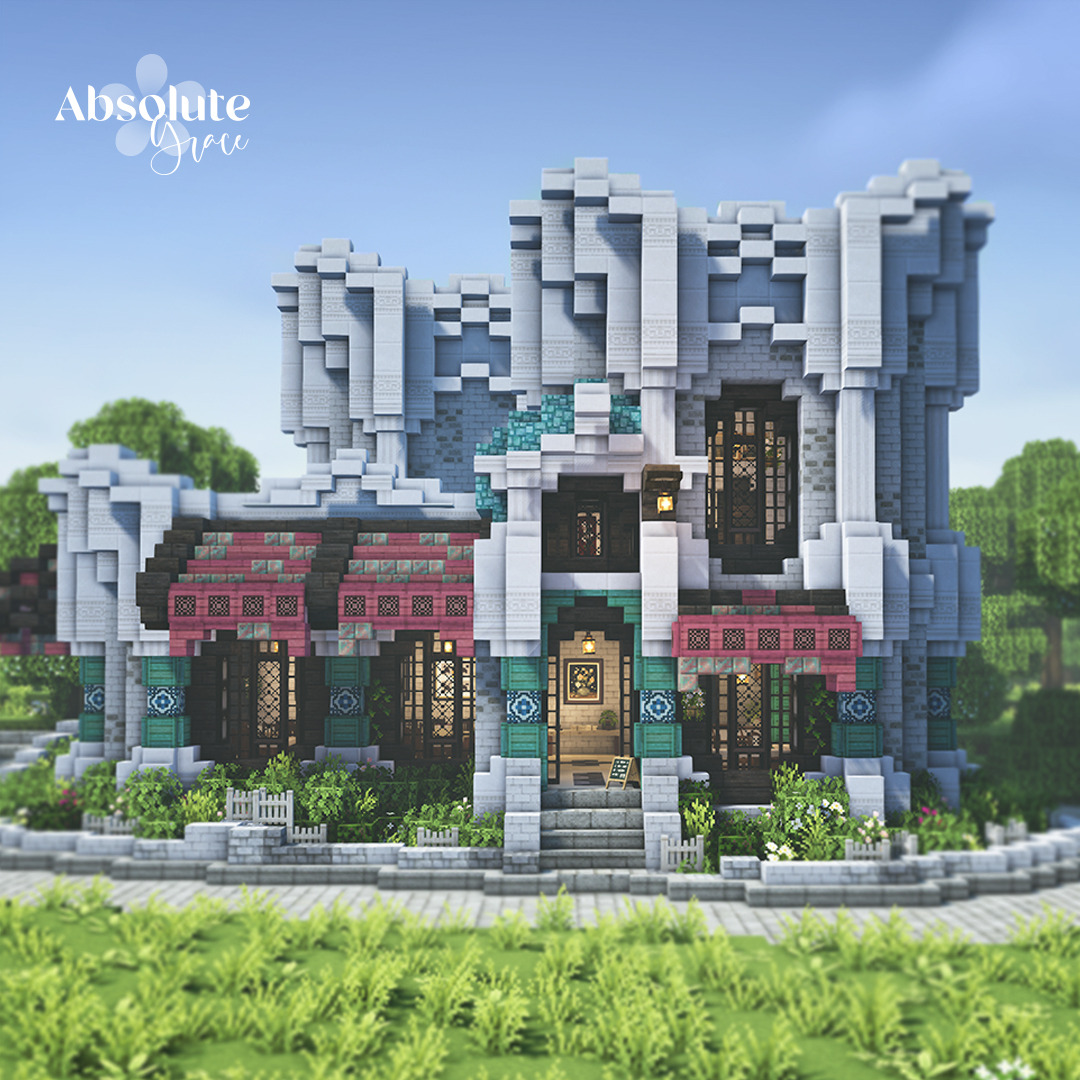The image is a digitally rendered, pixelated artwork of a grand, castle-like building set against a clear blue sky with no clouds. The top left corner of the image features the text "absolute grace." The majestic structure, which resembles an elaborate house or castle, is predominantly gray and blue, with accents of red, green, and bronze. The building is constructed from various materials, including white stone and red brick. It has numerous windows and an ornate wood-bronze front door. The architectural design includes elegant columns and steps leading up to the entrance.

In the foreground, there's a neatly maintained green lawn with a white concrete pathway directly in front of the building. Surrounding the pathway is additional green grass and some plant life. Behind the building, pixelated trees can be seen, contributing to the serene and picturesque setting.